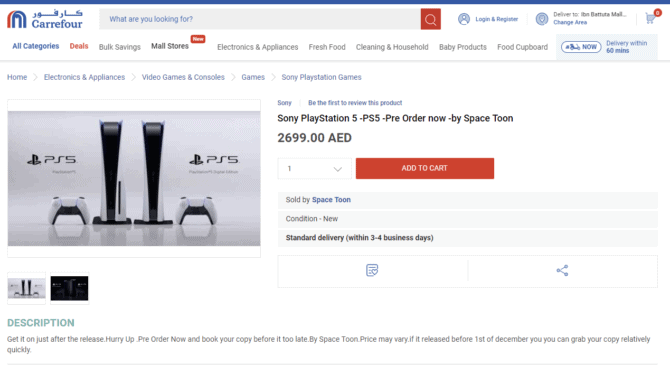The online image is from CARREFOUR, with the brand logo prominently displayed in the upper left-hand corner. Adjacent to the logo is a search bar inviting users to narrow down their search with the prompt, "What are you looking for?" To the right of the search bar, there is an account section featuring options to log in or register, represented by a circular icon.

Beneath the account options, there is a menu bar with several categories: 
- **All Categories**
- **Deals** (highlighted in red)
- **Bulk Savings**
- **Mail Stores** (marked with a red "new" banner)
- **Electronics & Appliances**
- **Fresh Food**
- **Cleaning & Household**
- **Baby Products**
- **Food Cupboard**
- **Deliver Now** (with a note indicating delivery within 60 minutes for same-day service)

Further down, there are additional tabs focused on specific interests:
- **Home**
- **Electronics & Appliances**
- **Video Games & Consoles**
- **Games**
- **Sony PlayStation Games**

The focal point of the image is a Sony PlayStation 5 (PS5), available for preorder through Space Tune, priced at $2,699.